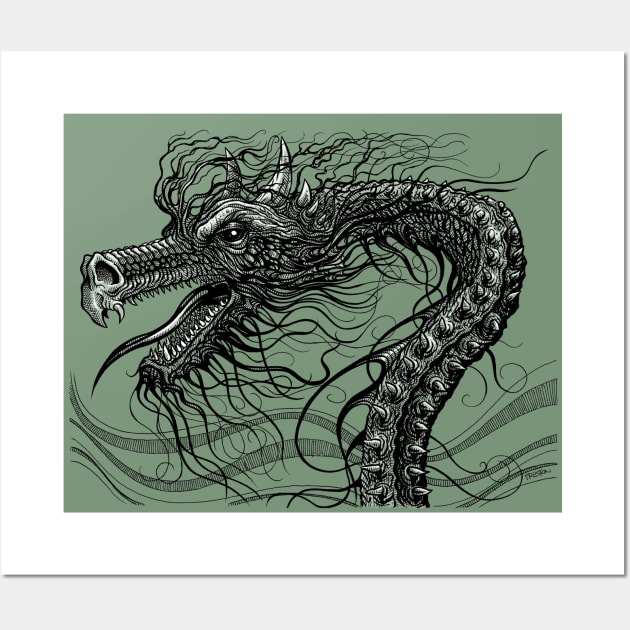This is a striking pen-and-ink drawing of an Asian-style dragon, intricately detailed and evocative of Japanese or Oriental art. The dragon is depicted in black ink on a light olive green background, which is framed by a white mat set against a slightly gray backdrop. The dragon's head is shown in profile, facing left, with an open mouth revealing sharp, white fangs on both the upper and lower jaws, and a long, pointed tongue extending outward. Its snout is long and scaled with a downward-hooked wide-nostriled nose. The eye is black with a pin light at its center, and it has a heavy, scaled eyebrow. 

From its head, long tendrils or wispy black fibers, possibly hair, flow upward and backward, stretching up from the crown, while two white horns rise from the crown where ears might be expected. Additional white horns decrease in size down the jawline. The dragon's serpentine neck curves elegantly from the base of the head, wrapping around to the right and twisting downward vertically. The neck is adorned with scaly, spiky features and raised horns along its spine.

Towards the bottom of the image, behind the dragon, wavy green lines suggest the creature emerging from water. The beautifully detailed artwork is signed by the artist in the lower right corner, though the signature is not legible. Overall, the dramatic contrast between the olive background and the black ink drawing, combined with the meticulous detail, makes this piece exceptionally eye-catching.